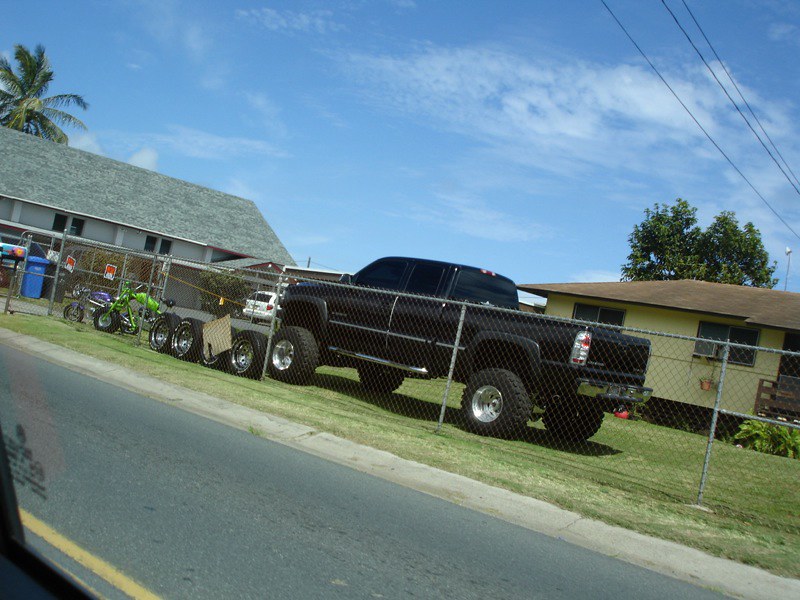This photograph, seemingly taken from the side window of a moving vehicle, showcases a front yard with a prominent black pickup truck at its center. The truck, conspicuously elevated above its tires, features black wheels and possibly a chrome rear bumper. It is parked on closely shorn green grass, indicating it is likely on private property. A gray chain-link fence stands in front of the truck, hinting at the enclosed nature of the property. Beyond the truck, a single-story yellow house with black trim is visible to the right. Against the fence, four large spare tires are lined up with a cardboard sign suggesting they might be for sale. Nearby, two motorcycles—a lime green one and a blue one—also have signs, though they are too distant to read. To the left sits a two-story building with white siding and a gray roof, with a white minivan parked in its driveway. The sky above is vivid blue with scattered white clouds, and the foreground includes a blacktop road with yellow lines, adding to the dynamic composition of the scene.